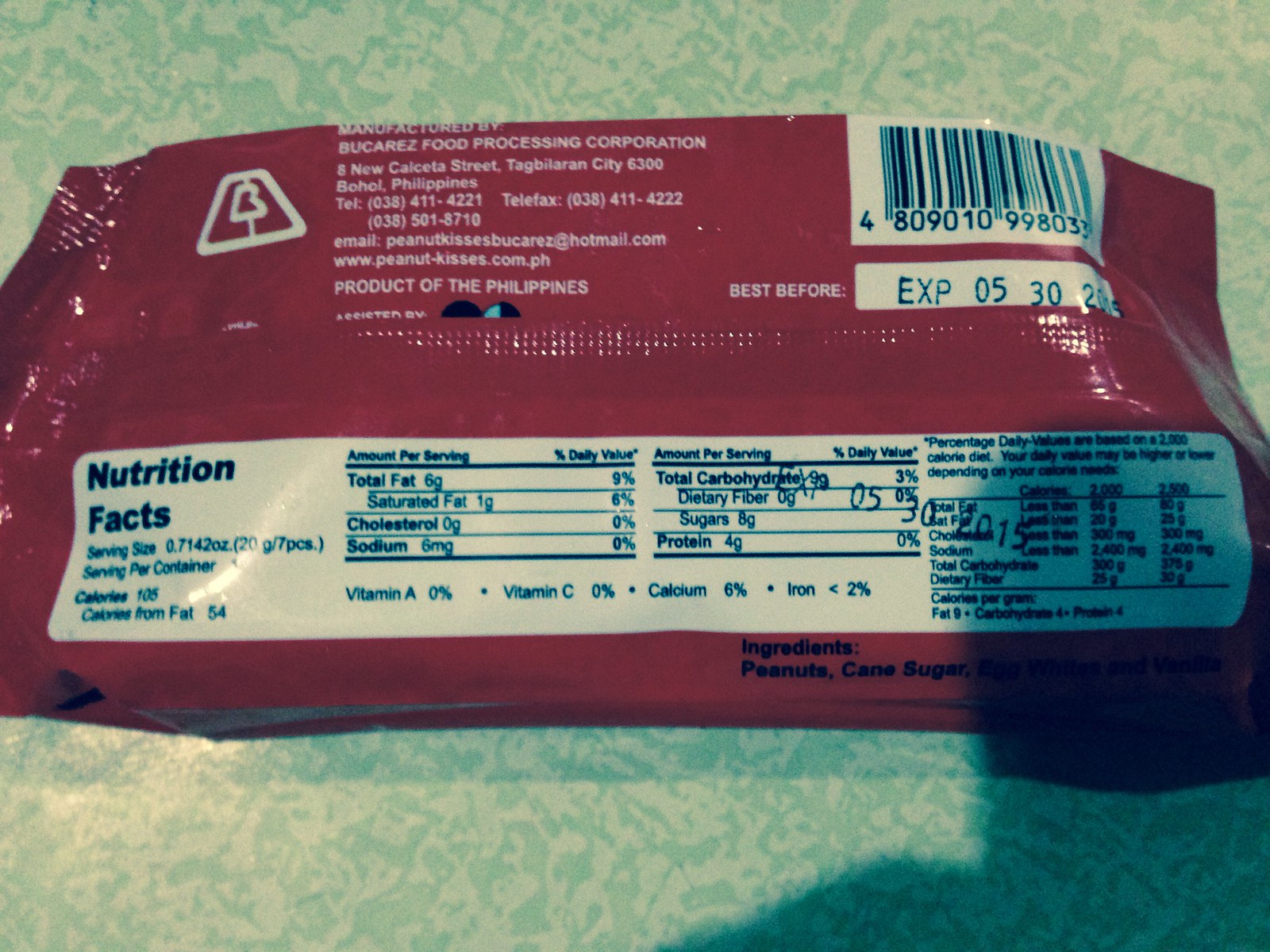The image depicts the back of a product wrapper, predominantly colored in red. At the top of the wrapper, there is a barcode. The expiration date is listed as "May 30," although the final digit of the year is unclear and could be either '21 or '24. Below the barcode, there is a white rectangular section containing nutritional facts, which are written in blue text. The wrapper indicates that the product contains 125 calories. Additional text on the red background describes the ingredients and production details, all in white font. It's noted that the product is made in the Philippines, and there are phone numbers provided for customer inquiries. A shadow of the person taking the photo is also visible across the table.